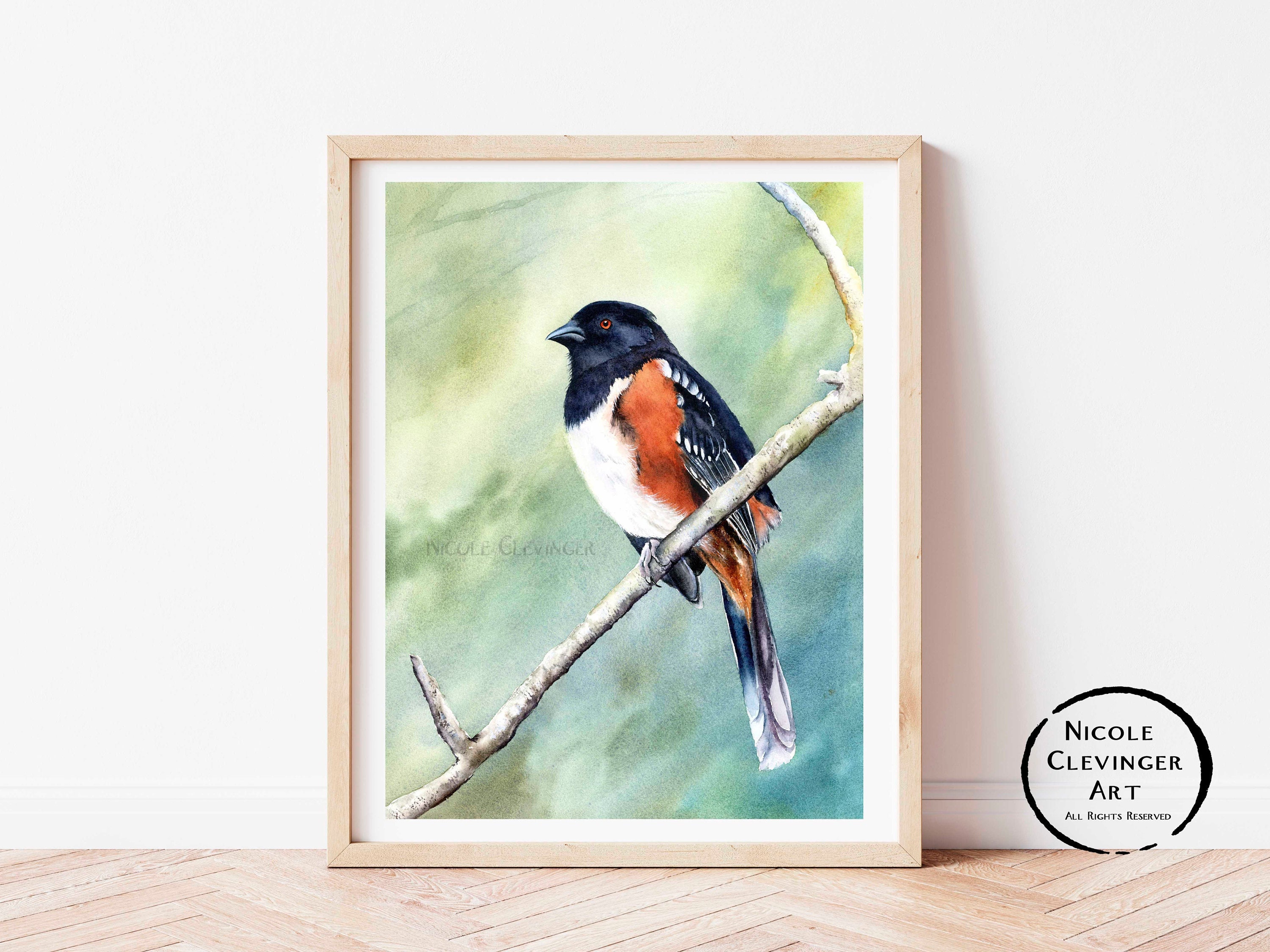A framed watercolor art piece by Nicole Clevenger is sitting on a wooden zigzag-patterned floor, leaning against a very white wall with crown molding trim visible in the bottom right corner. The painting is encased in a pink wooden frame with a half-inch white mat surrounding it. In the center of the artwork, a bird is perched on a branch that extends from the lower left to the upper right. The bird features a black beak, neck, head, and back that transitions into a bluish hue, an orange eye, a white belly, and an orange patch between its belly and wings. The background blends gradients of pastel yellows, greens, blues, and whites. The artwork is signed with "Nicole Clevenger Art, all rights reserved" in a black circle with a paintbrush effect, positioned in the bottom right corner. Additionally, the text "Nicole Clevenger" appears almost transparent to the left of the bird.